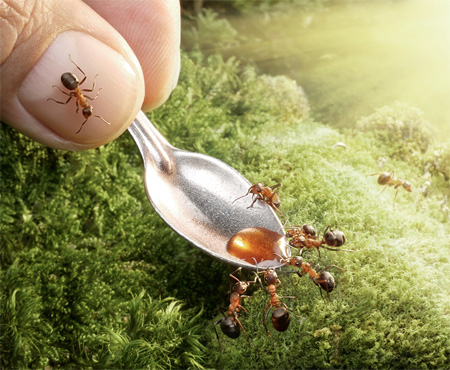The photograph captures a white hand, specifically the thumb and forefinger, holding a small, silver spoon filled with a sweet brown liquid, possibly honey. The scene is set outdoors, amidst a lush green area with bright sunlight streaming in from the top right corner. Multiple ants are visible, with five clustered at the edge of the spoon, seemingly attracted to the liquid, and one ant perched on the thumb. Another ant is on the spoon itself, and a single ant can be seen in the background walking away on the greenery. The hand and spoon take up the top left corner of the image, emphasizing the tiny, detailed interactions against a vibrant, sunlit backdrop.